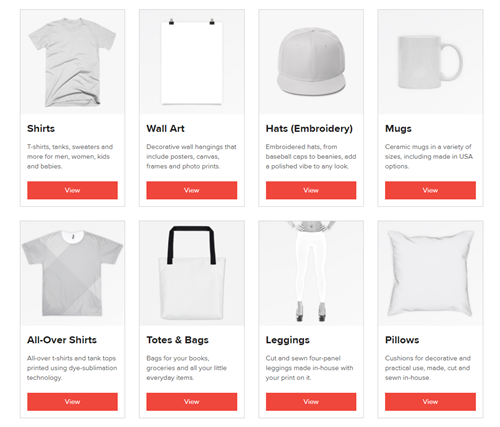The image depicts a personalization-focused website with a sleek, predominantly white interface accentuated by black text and red action buttons. The homepage showcases eight categories for customizable items:

1. **Apparel**: The first item featured is a plain white T-shirt. The description mentions a variety of garments available for personalization, including shirts, tanks, sweatshirts, and more for men, women, kids, and babies. A red "View" button is available for more options.
   
2. **Wall Art**: This section offers various decorative wall hangings like posters, canvas prints, framed art, and photo prints.
   
3. **Hats and Embroidery**: Illustrated by a hat, this category includes a range of embroidered headwear options, from baseball caps to beanies, designed to add a polished vibe to any look.
   
4. **Mugs**: A selection of ceramic mugs in various sizes, including options made in the USA.
   
5. **All-over Shirts**: This section features shirts and tanks that are printed using advanced dye sublimation technology for full-coverage designs.
   
6. **Totes and Bags**: A variety of bags designed to carry books, groceries, and other everyday items.
   
7. **Leggings**: Custom-designed, cut-and-sewn four-panel leggings made in-house with your personalized print.
   
8. **Pillows**: Cushions that can be used both decoratively and practically.

The website is visually organized and highlights the versatility and breadth of customization options available.